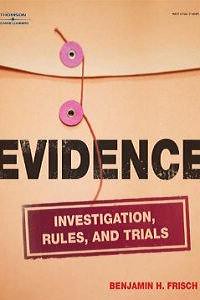The image is a low-resolution, small photograph that appears to depict a book cover. The cover resembles a brown manila envelope typically used for office correspondence, featuring a string closure rather than adhesive tape. Prominently centered on the cover is the bold black title "Evidence," with "Investigation Rules and Trials" beneath it in a large red label that resembles a stamp, giving it a formal and authoritative look. The author's name, Benjamin H. Frisch, is also present. The overall design evokes a confidential or top-secret dossier, enhancing the investigative theme of the book.